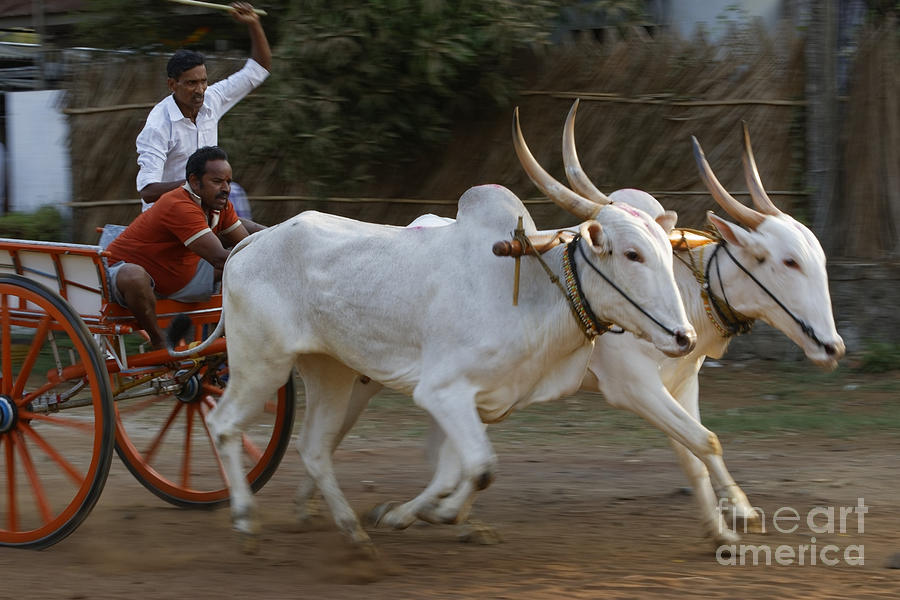This is an action-packed photograph capturing two large white oxen with curve-back brown horns featuring black tips. These oxen, moving at high speed and slightly blurred, are adorned with black straps over their noses and necks and are yoked to a wooden rod. They are pulling an open-top cart with orange spoked wheels and rubber tires, featuring a white body with orange framing. Two dark-skinned men with mustaches and short dark brown hair occupy the cart; one in an orange shirt is seated and appears to be tugging on a rein, while the other, standing in a white shirt, holds a whip or cane above him, urging the oxen forward. In the background, one can spot a fence and trees, suggesting a rural setting possibly in India. Fine Art America’s watermark is visible in the bottom right corner, adding a touch of authenticity to this dynamic and candid moment.